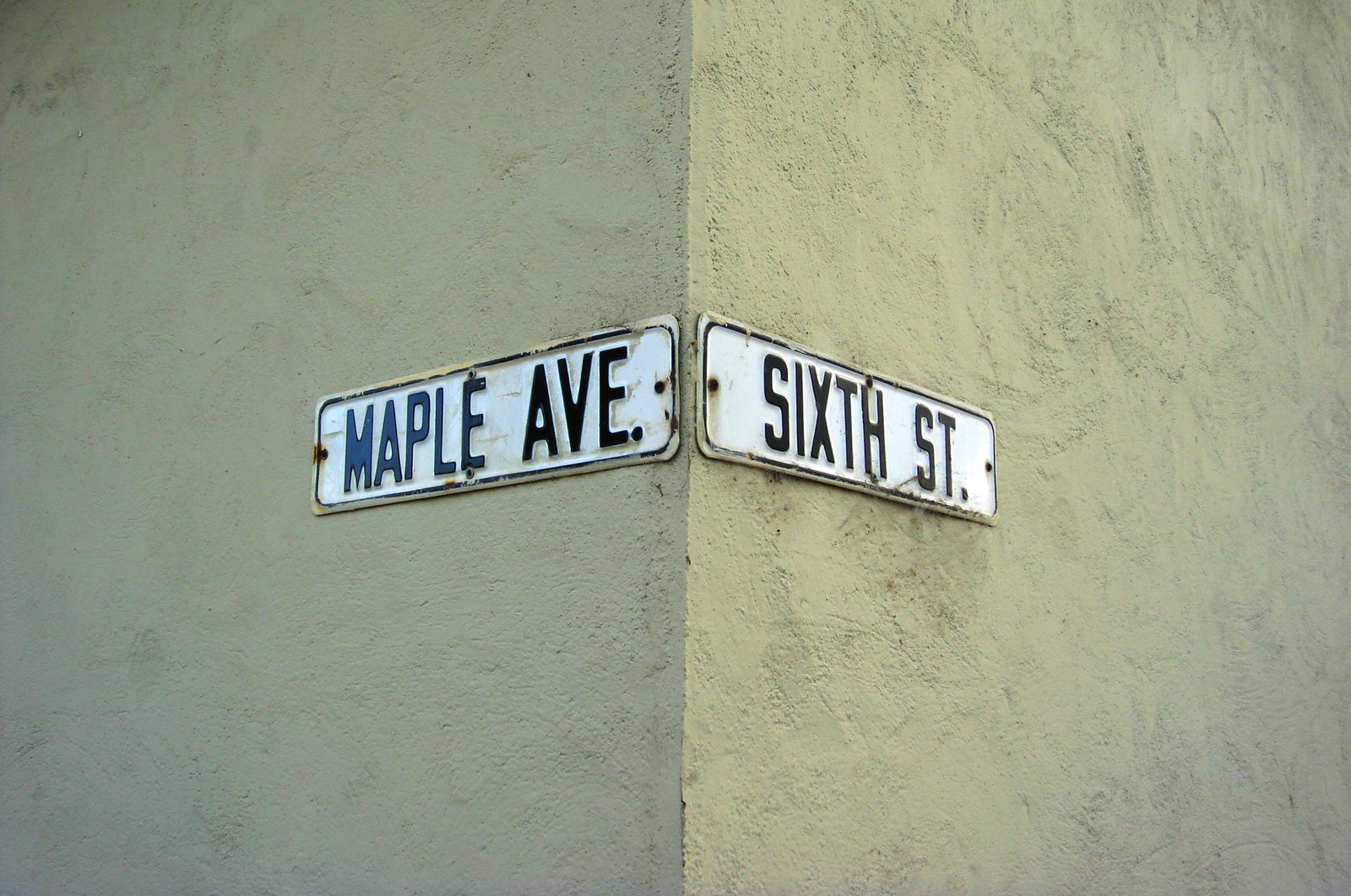A photograph taken outdoors during the daytime showcases the sharp corner of a building constructed from light tan, almost gray-colored stone. The building forms a very acute angle at the intersection, with two sides prominently displayed. Affixed to each wall are white street signs bordered in black, featuring bold black lettering. One sign indicates "Maple Ave," while the other reads "6th St." The overall composition captures the distinct architecture and provides clear details of the street signs, highlighting the location's specific intersection.